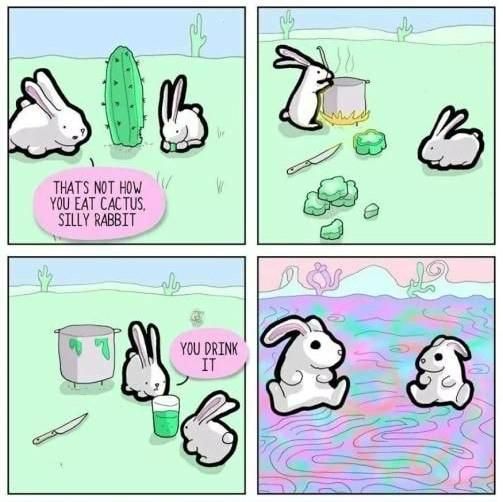This detailed, four-panel comic strip seems to reference a humorous and surreal experience involving two white rabbits and a cactus. 

**Panel 1:** Located in the top left, this panel features two white bunnies outlined in black, standing on either side of a green cactus in a green desert-like setting. One bunny, on the left, comments in a pink speech bubble, "That's not how you eat cactus, silly rabbit."

**Panel 2:** On the top right, the scene shows one bunny chopping up the cactus with a knife, while a pot boils on a fire next to them. The other bunny watches curiously.

**Panel 3:** In the bottom left panel, the cooked cactus has been transformed into a glass of green juice. The bunny with the knife instructs the other, "You drink it," as the curious bunny looks on.

**Panel 4:** The final panel, on the bottom right, depicts the two bunnies sitting down, seemingly under the psychedelic effects of the cactus juice. The landscape around them becomes a swirly, vibrant mix of purple, green, and blue hues, and their eyes are wide and dilated, suggesting a hallucinatory experience.